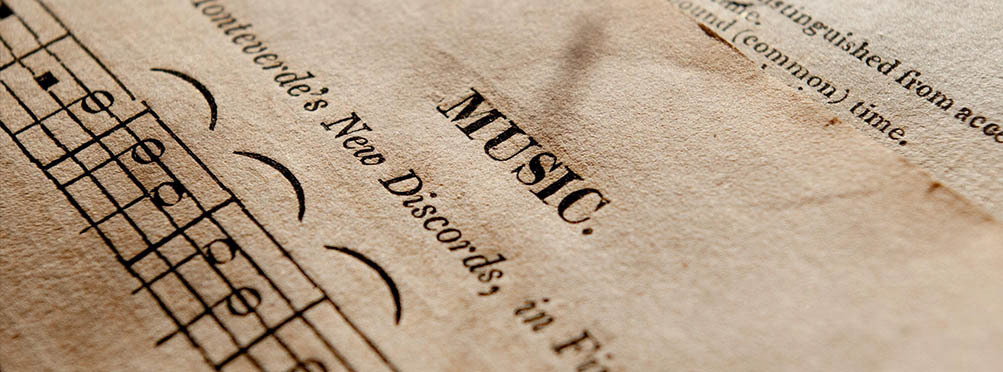The image displays a close-up, angled view of aged sheet music, giving it a light tan and off-white background. The main piece of paper is positioned diagonally from the upper left to the lower right. At the top-center in uppercase letters, it reads "MUSIC," followed by "Monteverdi's New Discords in F..." with the rest of the word cut off by the photo's frame. Below this title, there is a musical ledger (or stanza) with the traditional five horizontal lines and vertical bars. Specific musical notations are visible, including a small letter "P" with a long line and open circle, a solid black square note, and three arch-like symbols above the staff. In the upper right-hand corner, a second piece of paper partially peeks out from underneath, revealing fragments of text: "distinguished from A-C-C-O-U-N-D," with "common" in parentheses and the word "time." The photo is horizontally elongated, emphasizing the detailed inspection of this antiquated and slightly yellowed music sheet. The color palette consists primarily of shades of black, brown, and white.